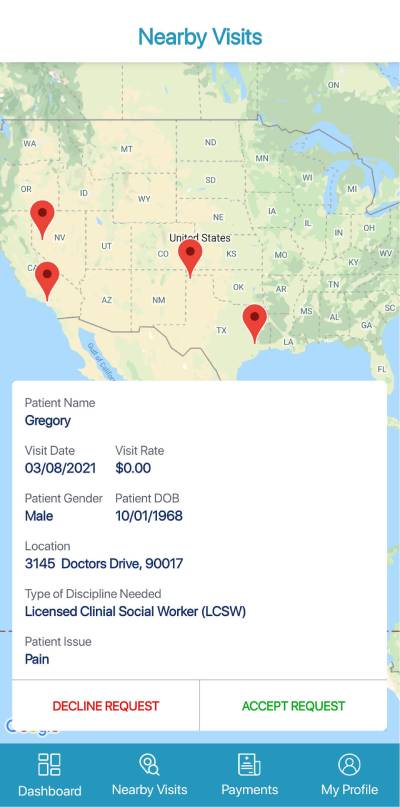The image appears to be a screenshot taken in portrait mode on a mobile phone. At the top of the screen, in blue text, it reads "Nearby Visits." Below this header is a map of the United States, featuring two-letter state abbreviations for each state and including parts of Canada. The map is detailed with state boundaries and is centered around the text "United States." There are four red markers indicating specific locations on the map: one in Nevada, one in Southern California, one in Northern Texas, and one in Southeastern Texas.

Beneath the map, there's a white information panel displaying patient details:
- **Patient Name:** Gregory
- **Visit Date:** 03/08/2021
- **Visit Rate:** $0
- **Patient Gender:** Male
- **Date of Birth:** 10/01/1968
- **Location:** 3145 Doctors Drive, 90017
- **Type of Discipline Needed:** Licensed Clinical Social Worker
- **Patient Issue:** Pain

At the bottom of the white panel, there are two buttons: a red "Decline Request" button and a green "Accept Request" button. Below this, there is a navigation bar in blue with options labeled "Dashboard," "Nearby Visits," "Patients or Payments," and "My Profile."